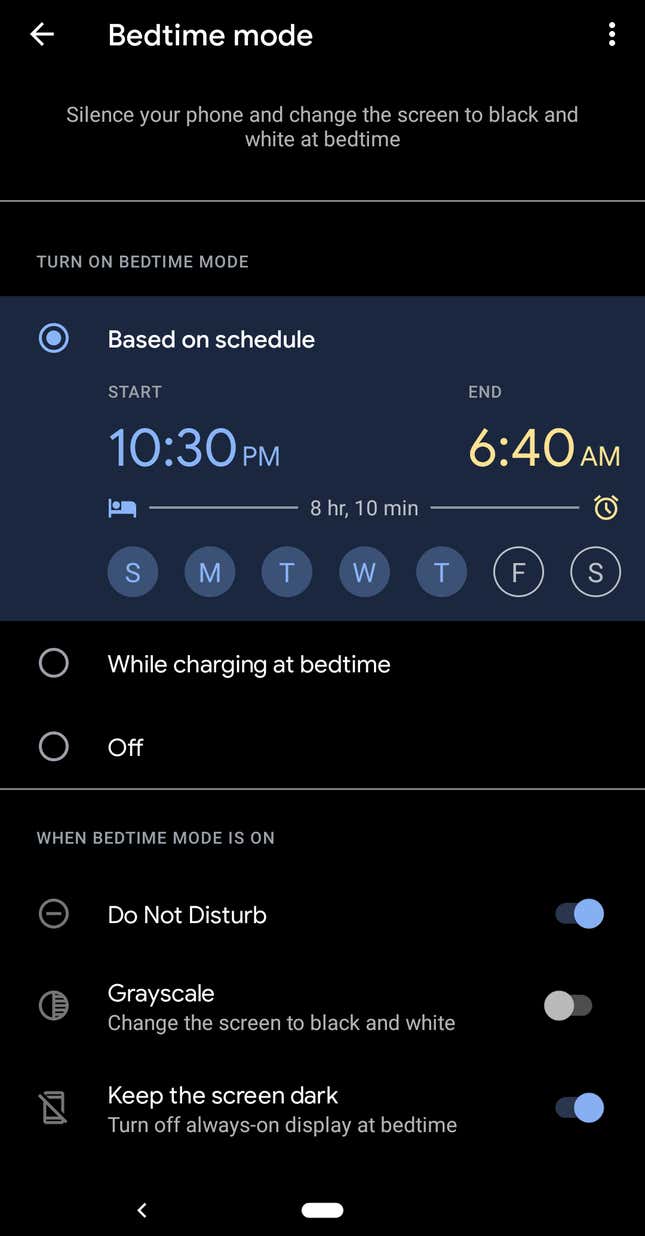The image is a screenshot from an Android phone's settings page, specifically showcasing the "Bedtime Mode" feature. Positioned in the top left corner, the page is prominently titled "Bedtime Mode." This feature appears to allow users to schedule a specific timeframe for Bedtime Mode activation, in this case, from 10:30 p.m. to 6:40 a.m. The purpose is to help manage phone usage during designated sleep hours.

The page details several customizable options available during Bedtime Mode, including:

1. **Do Not Disturb**: Silences calls, messages, and notifications.
2. **Grayscale**: Changes the display to black and white to reduce screen engagement.
3. **Keep the Screen Dark**: Dims the screen to minimize light disturbance.

Each option is accompanied by a slider on the right side, enabling users to toggle these settings on or off. The entire settings page features a sleek black background with white text for high contrast and easy readability. This screenshot effectively illustrates how an Android user can configure Bedtime Mode to promote better sleep hygiene by minimizing phone interaction during late-night hours.